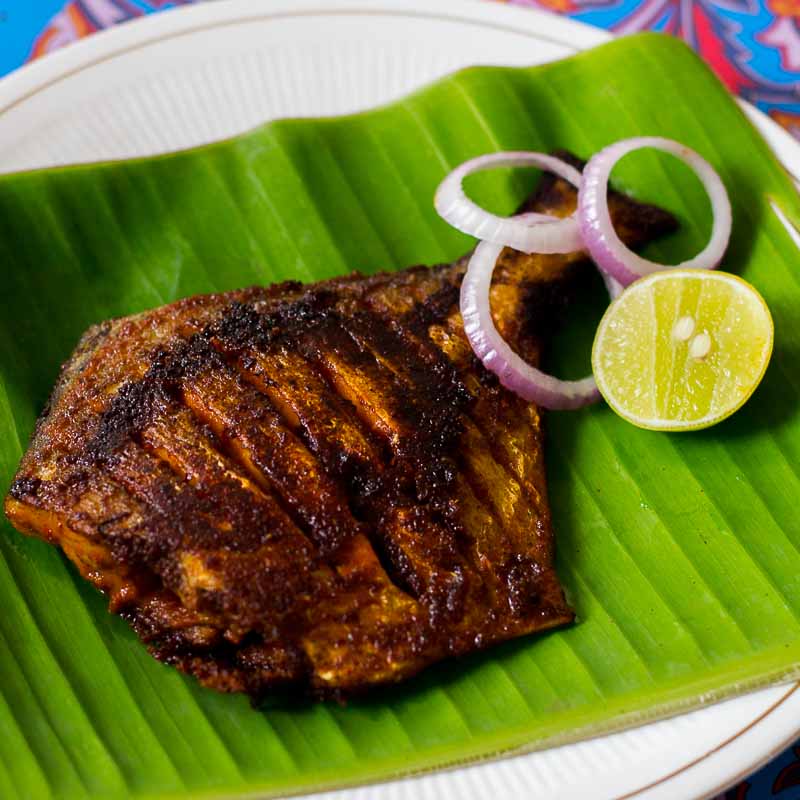This detailed image depicts a close-up view of a well-grilled piece of fish, characterized by its dark brown to blackened crispy exterior. The fish is garnished with three overlapping rings of red onion and accompanied by a visibly halved lime or lemon, with two seeds discernible within it. Serving as a bed for the fish is a green leaf, which rests atop a ridged white plate with a brown trim around its edge. The plate itself is set against a tablecloth adorned with blue, orange, and red designs, visible in the upper corners of the image.